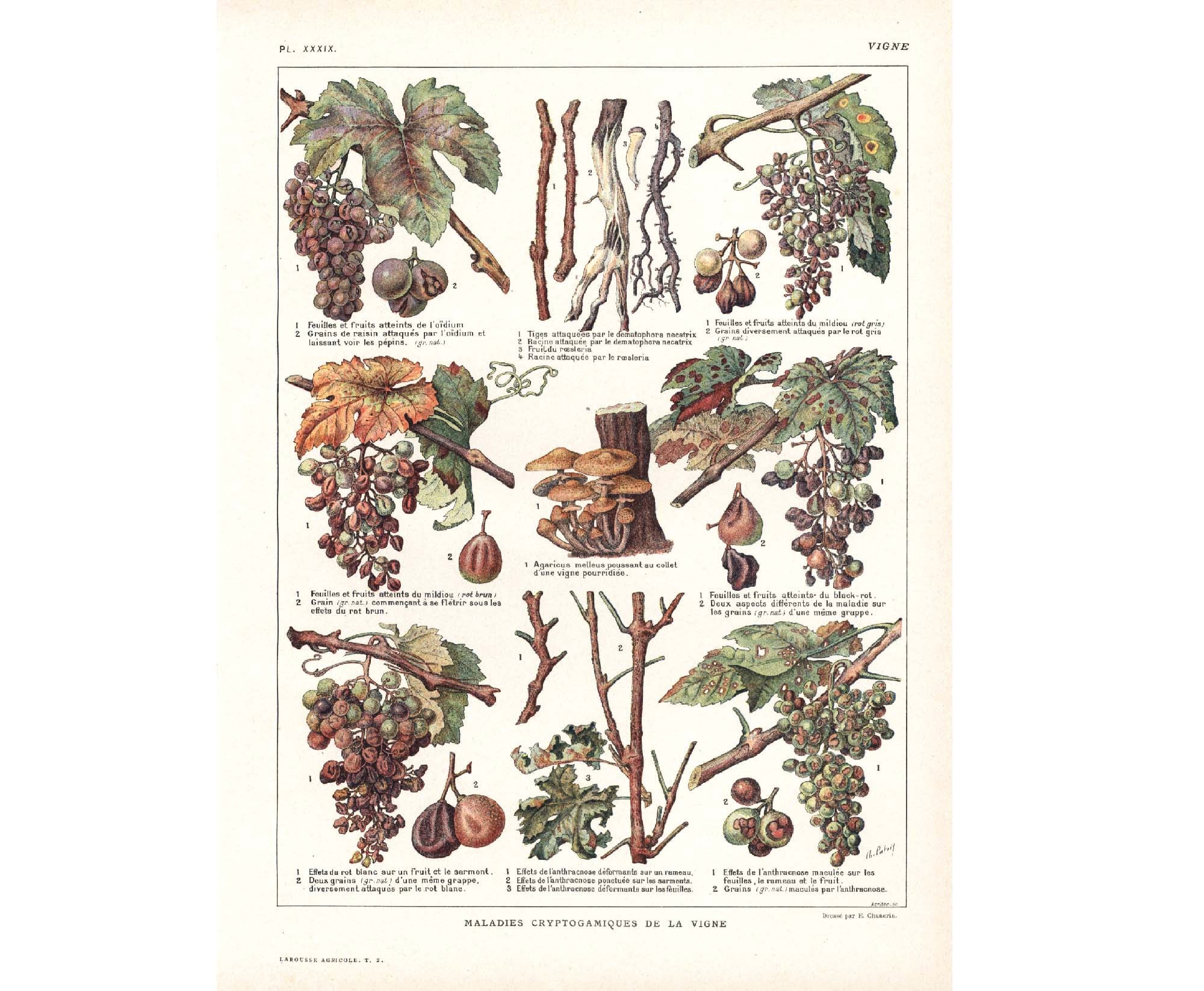The image appears to be an illustrative page from an aged book or science magazine, likely French, dedicated to showcasing various plants, particularly focusing on grapevines and their maladies. The top row features vivid color illustrations of grape leaves, branches, and bunches of both healthy and damaged red grapes. The middle section displays images of roots, a small stump with brown mushrooms, and various grape leaves, some bearing spots indicative of disease. The grapes shown range from plump and healthy to scrawny, green, and dried out, suggesting stages of decay or affliction. The bottom row presents a detailed progression of grape bunches, from healthy at the top to raisin-like and diseased at the base. Each image is accompanied by labels and descriptions in French, but they are too small to read clearly. The overall theme of the page appears to be related to the "Maladies Cryptogamiques de la Vigne," highlighting different fungal diseases affecting grapevines.